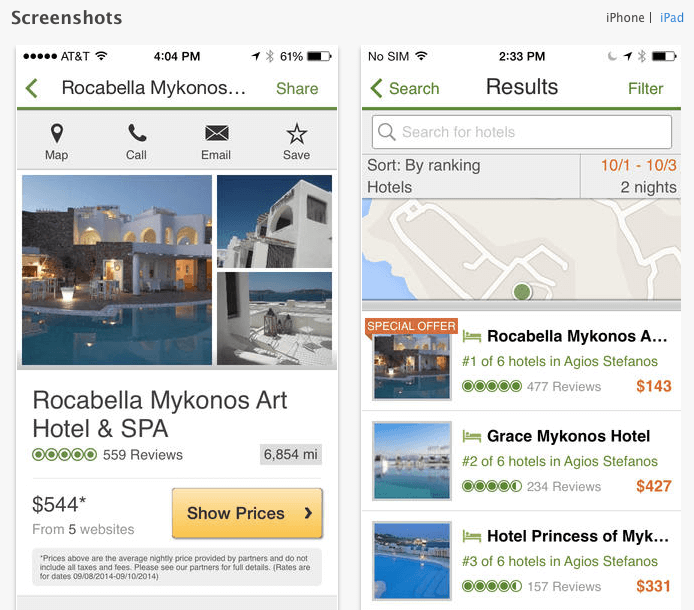This image is a composite of two screenshots on a gray background. In the top-left corner of the background, the word "screenshots" is displayed in bold black font, while the top-right corner features the words "iPhone | iPad" with the text "iPhone" in black and "iPad" in blue, separated by a vertical black line.

The left screenshot has a white background indicating a mobile phone interface. In the top-left corner of this interface, five black dots can be seen, followed by the text "AT&T," a Wi-Fi signal icon, the time "4:04 p.m.," and icons for location sharing, Bluetooth, a 61% battery indicator, and a battery icon. Below these status indicators is the text "Rockabella Mykonos" in black font, embellished with a left-pointing red arrow on its left and the red word "share" on its right. 

There is then a brown line demarcating the next section. This part features a gray rectangle containing four black icons: a location sharing icon labeled "map," a handset phone icon labeled "call," an envelope icon labeled "email," and a five-pointed star icon labeled "save." Below these icons are three images of what appears to be a luxurious white mansion or palace in Mykonos, complete with a large sun deck and pool.

The text below the images reads: "Rockabella Mykonos Art Hotel and Spa." It includes additional information that there are "559 room reviews" and the location is "6,854 miles away." A black line separates this text from the rest of the content.

Overall, this detailed and descriptive caption captures the essence and layout of the composite image, highlighting the specific elements contained within the left screenshot.